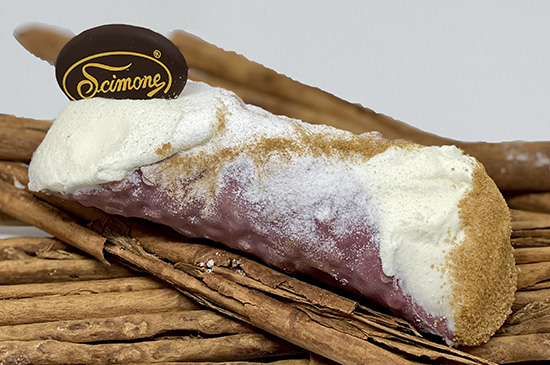This horizontally aligned rectangular close-up image captures a dessert that strongly resembles a cannoli. The cannoli is oriented diagonally with one end pointing towards the upper left, and the other end towards the lower right. The shell is partly covered with a white powdered sugar coating and dusted with a fine brown powder, likely cinnamon sugar. The right end of the cannoli features a profuse white cream filling, also dusted with cinnamon sugar, while the left end shows a solid white cream.

The cream at the left end is topped with a round, thin, dark brown chocolate disc that has a gold circle on the front and the word "Scimone" inscribed in gold print. The cannoli is resting on a surface made of narrow, cigar-shaped brown rods, possibly cinnamon sticks, accentuated with darker brown notches. The background of the image is a light gray, slightly blurred wall, providing contrast and focus to the intricate details of the cannoli.